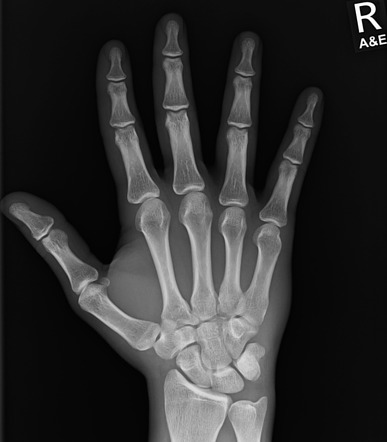This detailed x-ray image features a right hand, easily identifiable by the prominent letter "R" in the top right corner, accompanied by the smaller letters "A" and "E" beneath it. Set against a completely dark, black background, the x-ray reveals the intricate structure of the hand with striking clarity. The bones, displayed in white, stand out prominently, showcasing the alignment and detail of each finger, the wrist, and parts of the forearm. The hand appears to be held upright with fingers fully extended, displaying three distinct bone segments in each finger, connecting seamlessly to the bones in the palm and wrist. The skin's outline is somewhat translucent, adding depth and context to the skeletal structure. Notably, there appears to be some separation between the wrist bones and the arm bones, but no cracks or fractures are visible. The overall impression is that of a normal-sized hand, possibly belonging to a young person, suggested by the presence of wider areas at the end of the bones that could indicate growth plates.